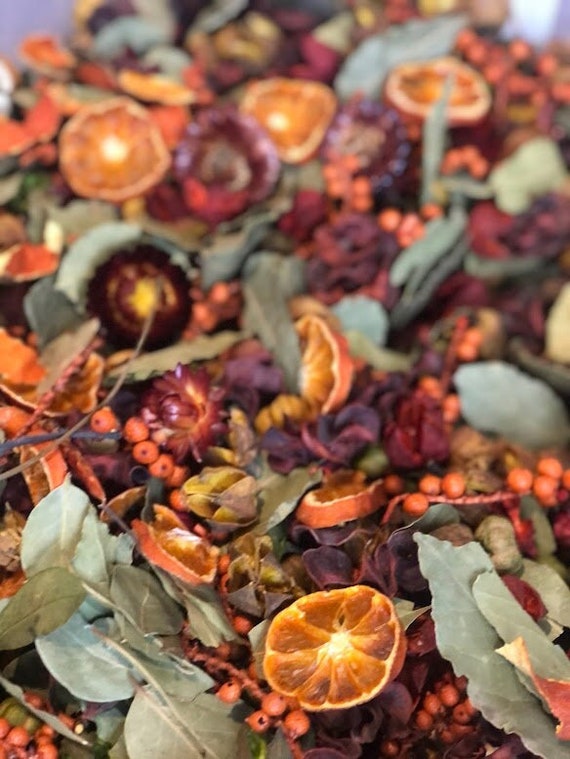This image is a detailed close-up of a vibrant potpourri mix, featuring a hodgepodge of dried fruits, leaves, seeds, and flowers. At the forefront are numerous mandarin or tangerine rinds, perfectly cut in half, showcasing their orange skins. These citrus halves appear dehydrated, suggesting some age. Scattered among these rinds are various green leaves, some intact, others torn, contributing to a diverse texture. Additionally, dark reddish-purple plant-like objects and small red and yellow flower bulbs, alongside tiny red flowers, are peppered throughout the composition. The background remains slightly out of focus, emphasizing the intricately mixed elements in the foreground, creating a visually rich and fragrant potpourri.